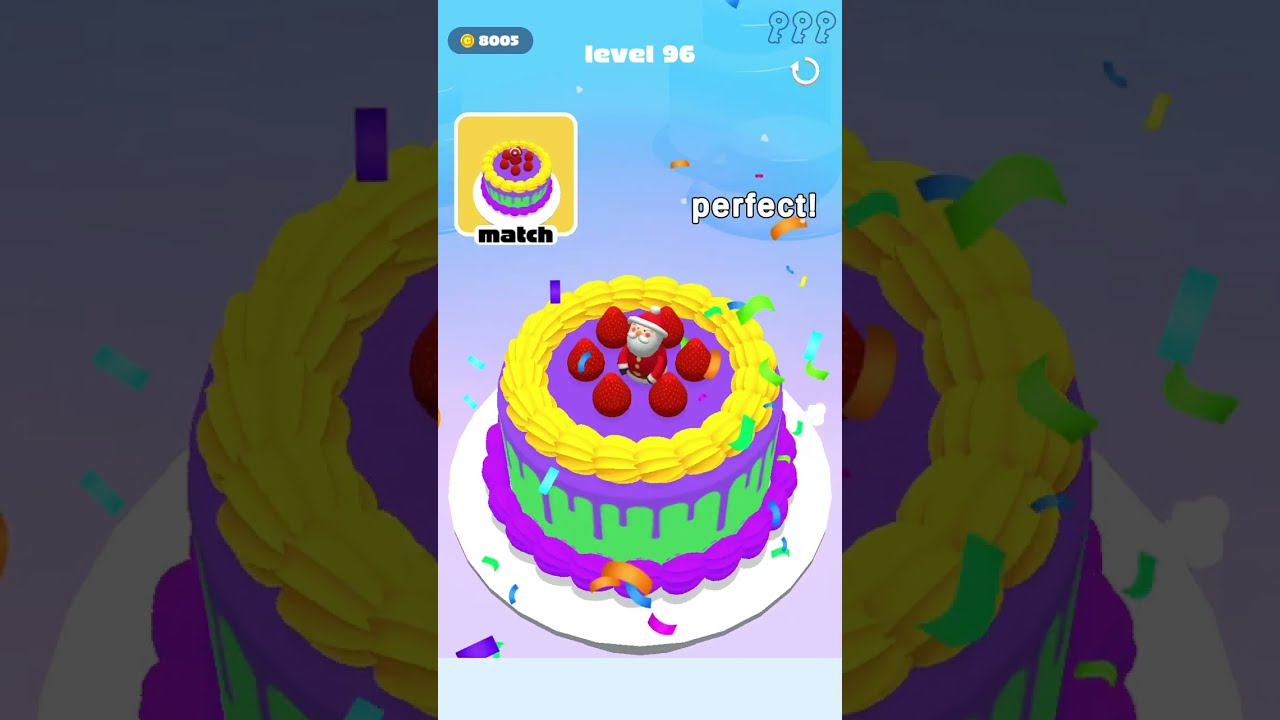The image features a cell phone screenshot of a match game set at level 96. The centerpiece of the image is a detailed cake, viewed from the top, adorned with a tiny Santa Claus toy dressed in a red hat and coat in the middle of upside-down strawberries. The cake is elaborately decorated with purple frosting, a circle of yellow frosting around the strawberries, and a pink frosting lining at the bottom. Confetti-like decorations in orange, blue, light blue, green, yellow, and purple sprinkle down the cake which sits on a white plate.

The overlaying game interface shows three hollowed-out key symbols outlined in purple at the top right, adjacent to a white "perfect" text. In the top left corner, there are gold coins amounting to 8,003. Below the keys, a white replay button is present. To the left, in a yellow box, is a slightly zoomed-out and mirrored image of the same cake, labeled "match" underneath. The game interface contrasts with a blue-and-purple gradient background that frames the whole display.